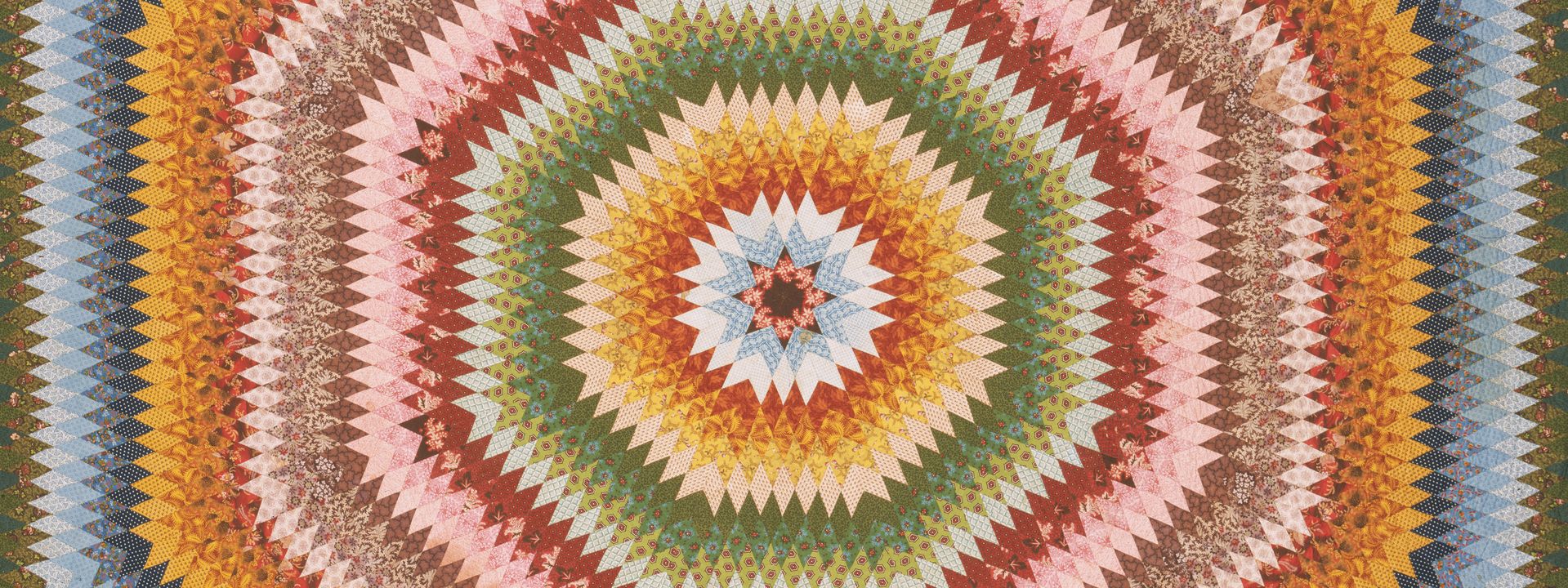This image is a close-up of a meticulously designed, multicolored quilt that appears almost as a photograph or digital painting. The quilt features an intricate, optical illusion-like pattern where layers of colors radiate from the center, creating a sense of movement. The central motif is a floral star surrounded by hexagonal and triangular shapes. Starting from the middle, the colors transition in concentric rings from light pink, to light blue, to white, to red, and then to yellow. Moving outward, the colors continue to vary, including shades of green, blue, orange, pink, and beige. Each layer grows larger and more complex, forming jagged, triangular edges that ultimately blend into vertical lines at the periphery. Distinct sections include multicolored dotted patterns and floral lines, with hues ranging from dark red to olive green and gravel gray. The entire quilt is composed exclusively of these colorful geometric shapes, creating a dynamic and visually engaging design.